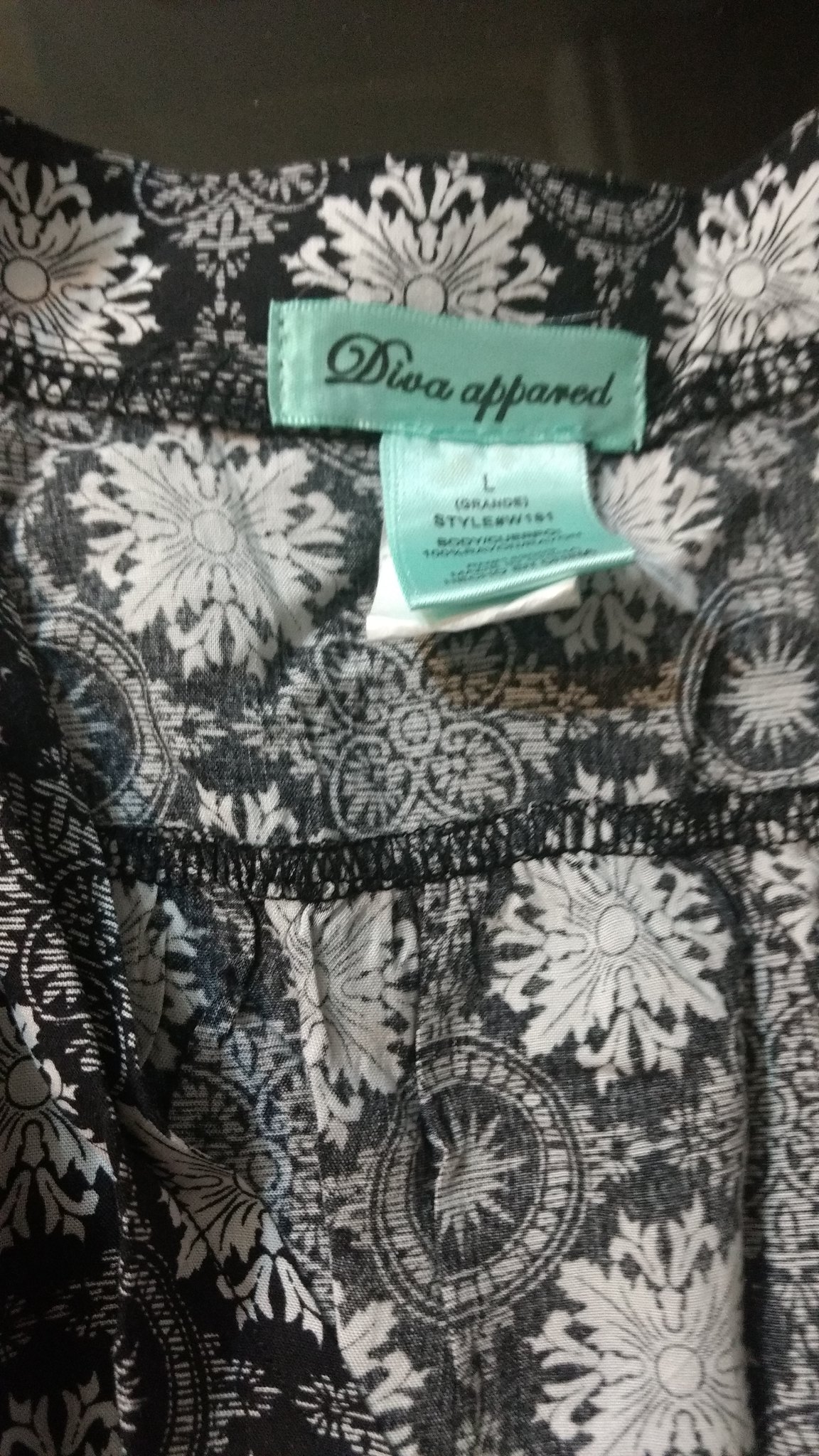This image features a detailed close-up of the inside of an article of clothing, specifically showing the tags stitched into the fabric. The garment itself is black with an intricate white floral design, and we can also see some black stitching. The teal-colored tags in the image exhibit a handwritten font, with one tag prominently stating "Diva Apparel." Beneath this, a second tag displays the size as "L" for large, along with the word "grande" in parentheses. There is also a notation of the style number, which appears to be "W 161." Additionally, there is a smaller, white tag below the others, which contains washing instructions. The exact type of clothing is indeterminate due to the close-up nature of the photograph, but the details give a sense of careful design and branding.